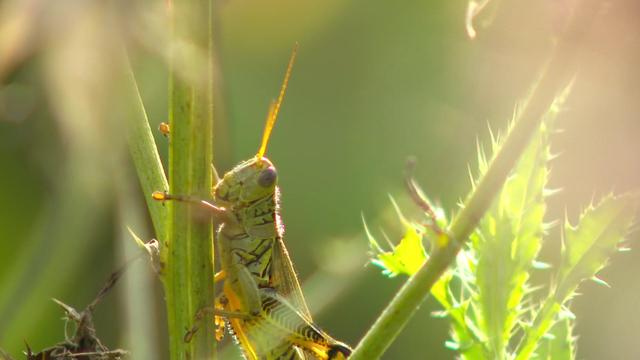The image is an outdoor photograph of a grasshopper clinging to a green plant stem under bright sunlight. The stem and the surrounding foliage give the entire scene a rich, green tone, enhanced by the blurred background with streaks of sunlight piercing through. The grasshopper, captured in a horizontal, rectangular frame, appears to be looking directly at the photographer. Its body is greenish-yellow with brown stripes and pronounced black eyes. It has an oval-shaped head and both its front and back legs can be seen gripping the stem. The leaves on the plant are prickly, adding texture to the vivid, green-dominated composition.